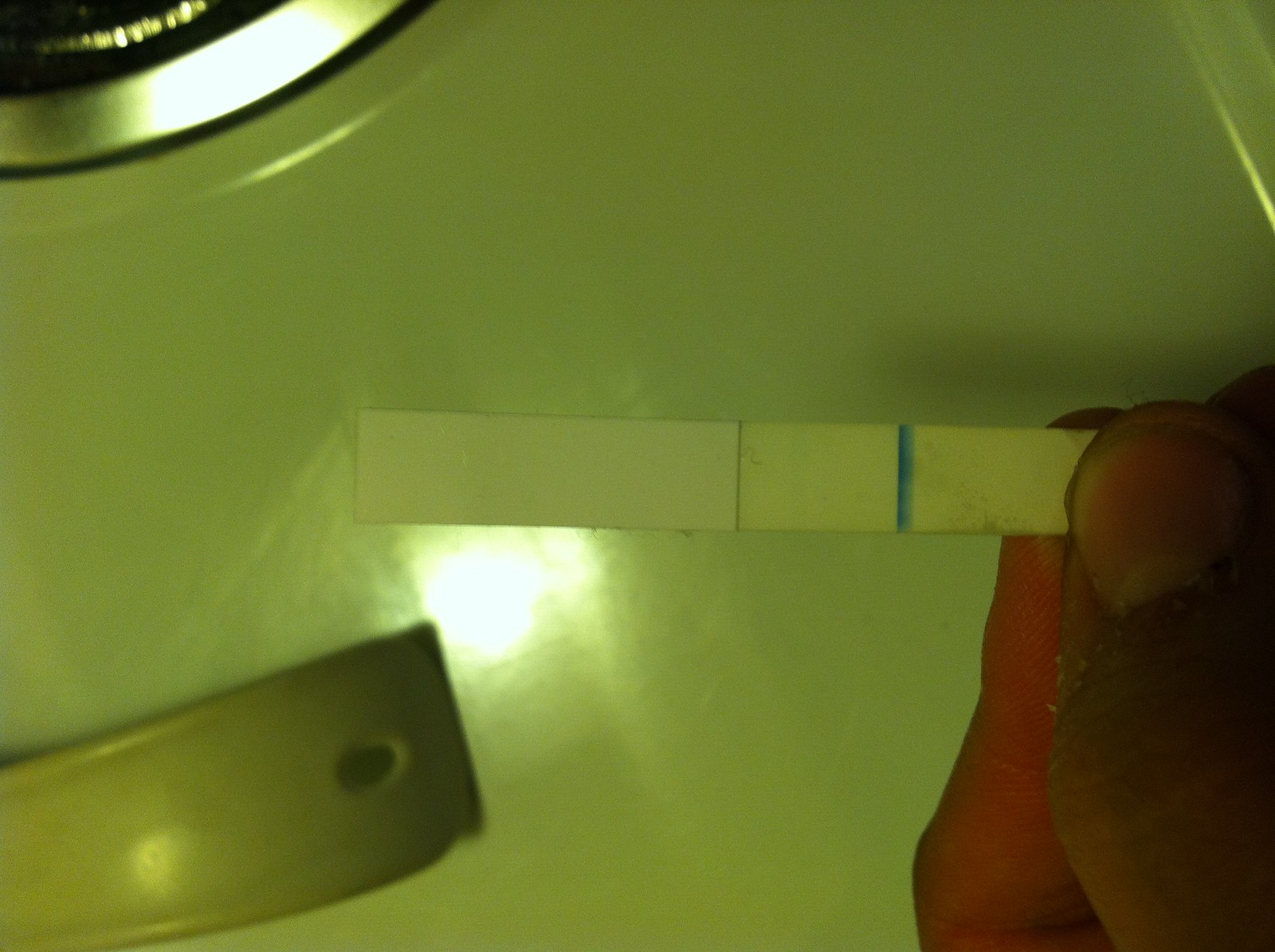The image depicts a close-up of three fingers from a hand holding a strip, which seems to be a pregnancy test strip. A prominent bright blue line on the strip suggests a positive result. The hand is positioned above a sink; part of the silver drain is visible, although much of it is obscured. Beside the sink, a mysterious metal object with raised ridges and an oval-shaped hole is present, though its exact purpose is unclear. Ambient light reflects off the sink, possibly from the ceiling above. The hand, which could belong to either a man or a woman, has nails cut very short, without any nail polish. The thumb displays rough, damaged skin, while the adjacent finger appears reddish, indicating a tight grip on the strip.